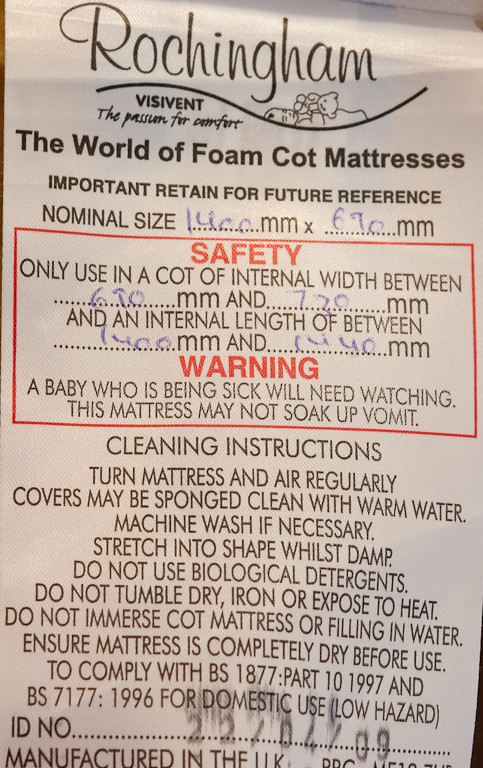This is a tall, rectangular image depicting a label, likely from a mattress, in white with a textured appearance and a slight bend at the top. At the very top, in black fancy font, it reads "Roshingham" with a curly underline and an image of a baby holding a teddy bear. Below this, it states "The world of foam cot mattresses" and includes the phrase "Important: retain for future reference."

Further down, the label lists a "Nominal size" in millimeters, with specific measurements filled in with blue pen: "1400mm x 670mm." Below that, a red rectangle with bold red letters reads "Safety Warning." In between these words, additional black lettering provides critical information. For safety, it notes: "Only use in a cot of internal width between 670mm and 720mm and an internal length of between 1400mm and 1440mm." 

For warnings, it mentions: "A baby who is being sick will need watching; this mattress may not soak up vomit." Cleaning instructions advise: "Turn mattress and air regularly; cover may be sponge cleaned with warm water; machine wash if necessary. Stretch into shape while damp. Do not use biological detergents, tumble dry, iron, or expose to heat. Do not immerse the cot mattress or filling in water. Ensure the mattress is completely dry before use."

At the very bottom of the label, there are compliance notations: "To comply with BS 1877, part 10, 1997 and BS 7177, 1996 for domestic use (low hazard)." Additional details include a final note or possibly an ID number.